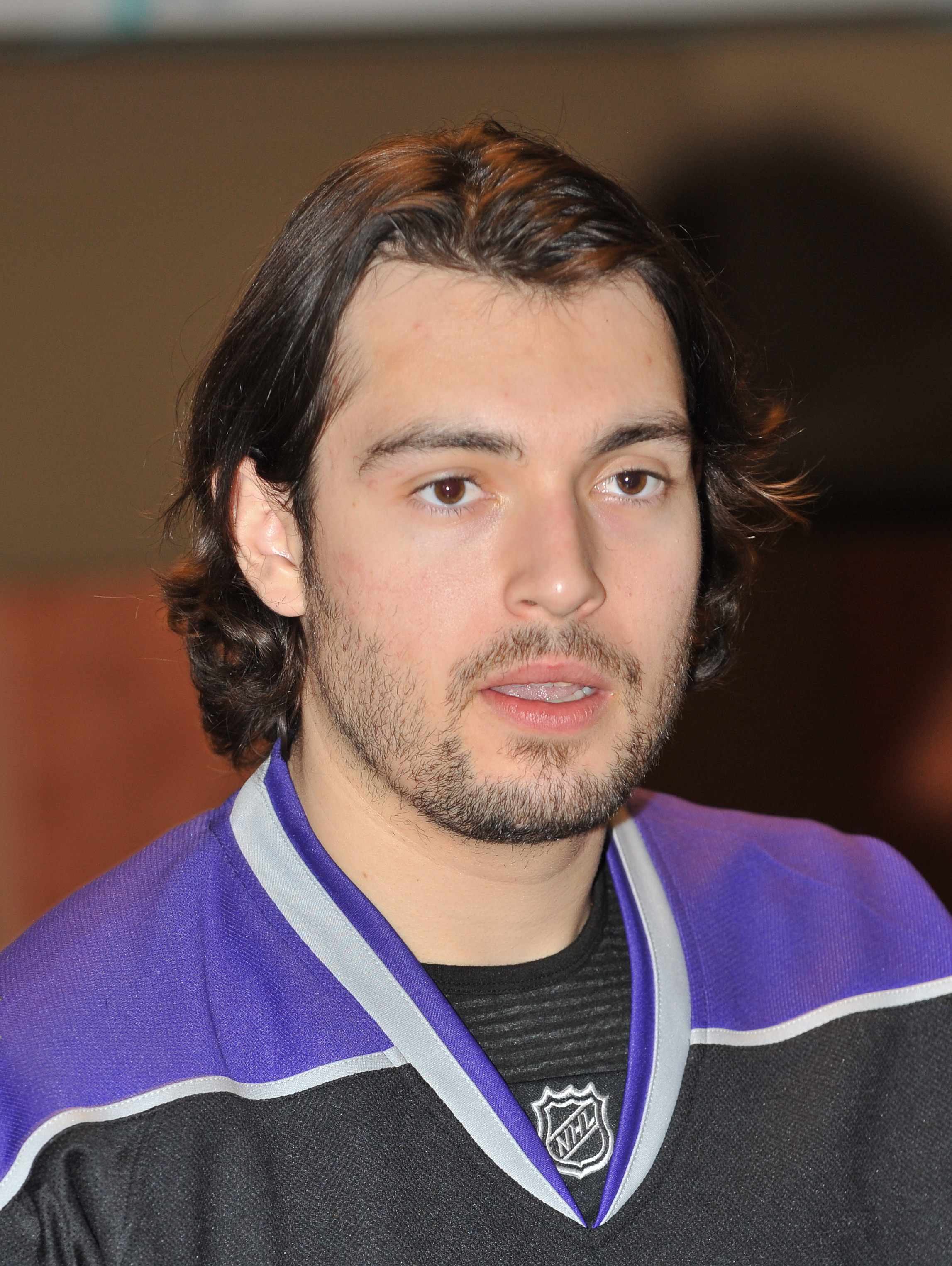In this indoor photo, the central figure is a man who appears to be a hockey player, as indicated by the NHL logo just below his neckline. He has dark brown, neck-length hair that appears slightly shaggy, and his facial hair consists of thin brown stubble that connects around his lips and under his chin. His brown eyes are focused forward, and his mouth is slightly open, as if he might be speaking. 

He is dressed in a distinctive hockey uniform, predominantly purple at the shoulders with black below, separated by a white line. The collar of the uniform is also marked by white and purple lines. The background of the image is blurry, featuring a mix of reddish and brown hues, with the left side appearing lighter due to his shadow. There is no clear indication of other people in the background, focusing all the attention on the man in the center.